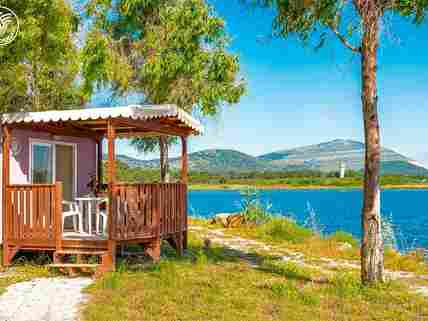The image is a small, vertically oriented, low-resolution photograph, possibly pixelated or degraded, depicting a picturesque scene by a lake. In the foreground, there is a quaint hut or cabin with a pink or reddish wall and a large glass door. The cabin features a brown wooden porch with white, ruffled coverings and white lawn furniture, including a table and chairs. Steps lead up to this cozy porch. Near the cabin, a light brown walkway meanders through green and brown grass. The background showcases a bright blue lake with serene water, bordered by rolling green hills or large mountains, some with granite facets. The scene is complemented by a vivid blue sky overhead and at least three trees, one prominently situated. The composition and elements suggest the season might be spring or summer, adding to the charm of this lakeside retreat.